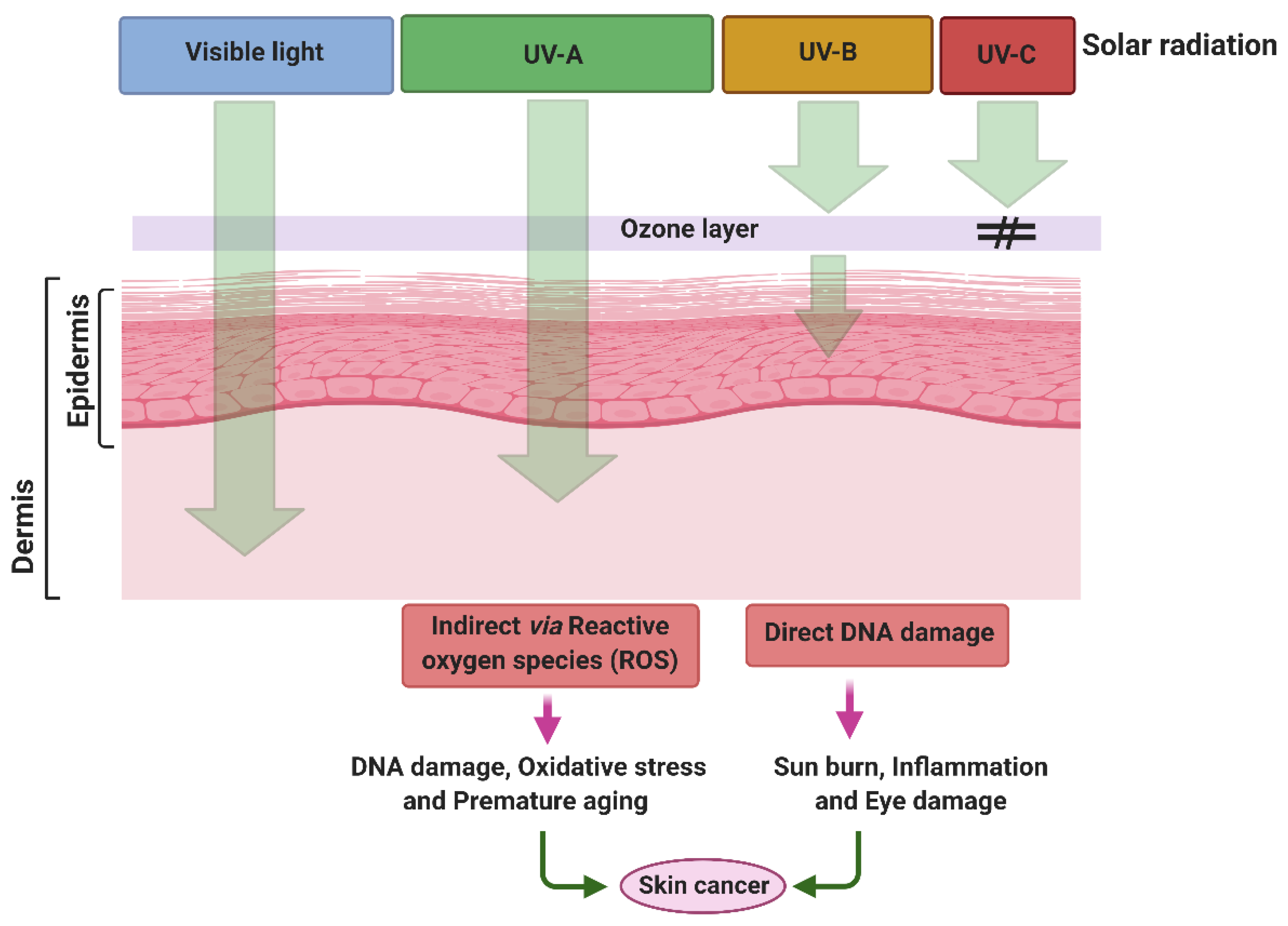This detailed educational illustration demonstrates how different types of solar radiation penetrate the skin. At the top, there are four labeled boxes from left to right: visible light (blue), UVA rays (green), UVB rays (yellow), and UVC rays (C). These are followed by a "solar radiation" label to the right. Below this, arrows indicate the depth of penetration through the ozone layer, epidermis, and dermis layers of the skin.

Visible light reaches all the way through to the dermis, the inner layer of skin, while UVA rays penetrate just into the dermis. UVB rays stop at the epidermis, the outer skin layer, and UVC rays are blocked by the ozone layer.

Accompanying these arrows, explanatory text describes the mechanisms of damage: "indirect via reactive oxygen species (ROS)" and "direct DNA damage." Arrows pointing downward further elucidate effects such as DNA damage, oxidative stress, premature aging, sunburn, inflammation, and eye damage, all ultimately leading to skin cancer, prominently illustrated in an oval at the diagram's bottom.